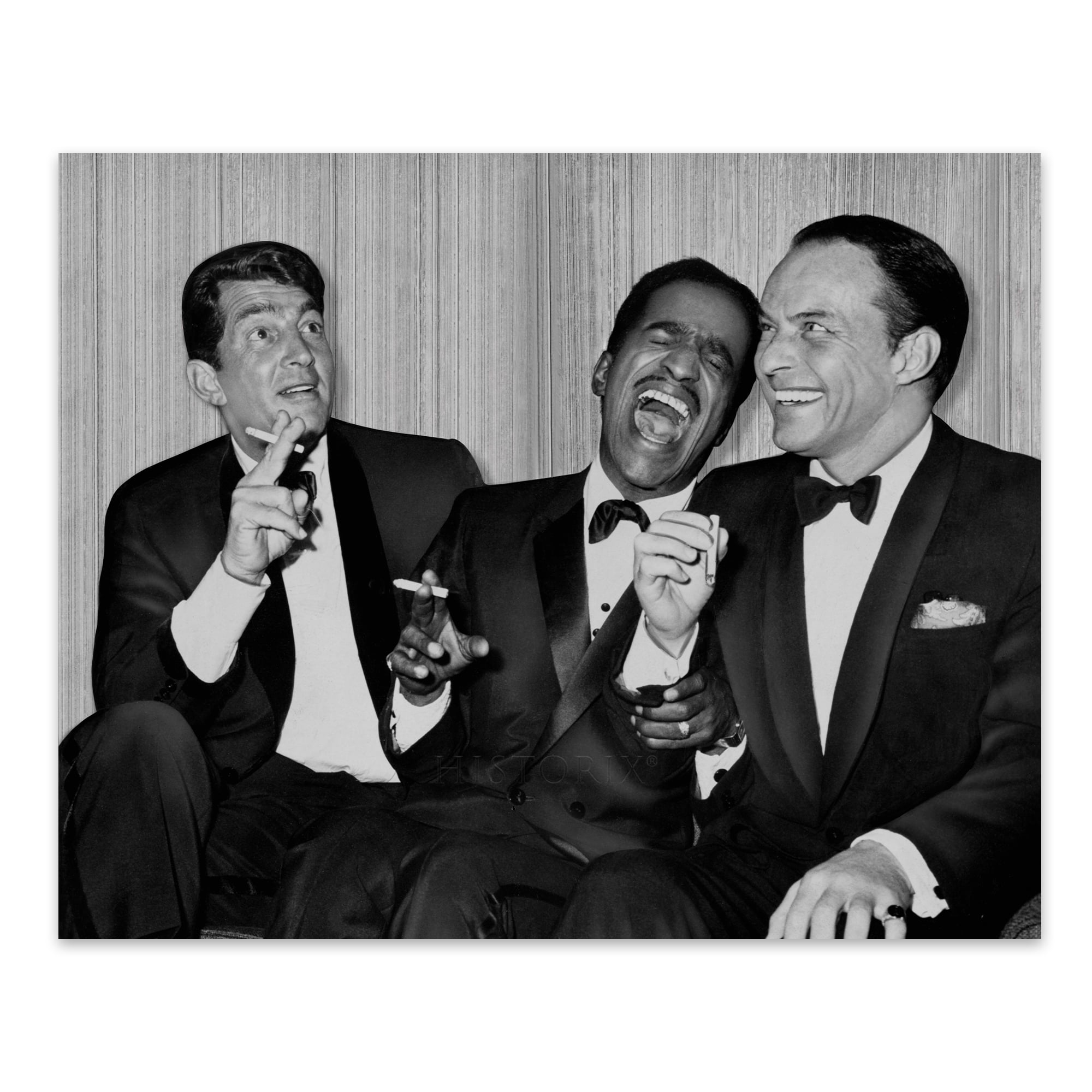This black and white photograph captures a vivacious moment from another era, featuring the iconic Vegas Rat Pack. On the left, Dean Martin, an Italian-American, is attired in a sharp tuxedo minus a tie, possibly with a bow tie hidden beneath his jacket. He smokes a cigarette, held casually with two fingers, and gazes upwards with a relaxed demeanor. In the center, Sammy Davis Jr., an African-American entertainer, is in the midst of a hearty laugh, his mouth wide open and eyes closed in sheer amusement. He clutches his cigarette between two fingers, his bow tie slightly askew, and his other hand gripping Frank Sinatra's arm. On the right, Frank Sinatra, identified as a Jewish man, completes the trio with his composed smile. He holds his cigarette delicately with three fingers and boasts the neatest bow tie of the group, accentuated by a neatly folded pocket square. All three men, dressed impeccably in tuxedos with white shirts and black slacks, exude an air of timeless elegance and camaraderie, clearly relishing the moment together.